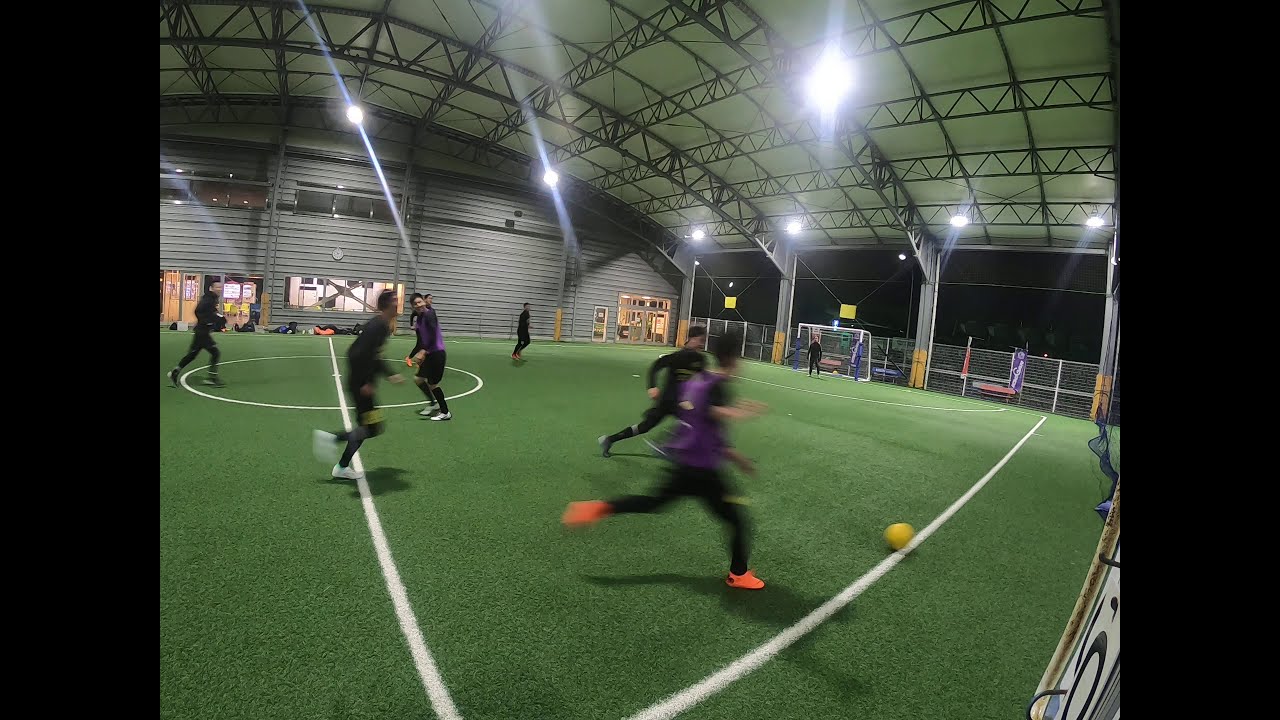In this photograph, we see an indoor soccer game being played on a field with green artificial turf, marked with white lines. The match appears to be a nighttime event, as indicated by the dark exterior visible through the open sections of the otherwise dome-shaped, well-lit stadium. The ceiling is adorned with fluorescent lights, casting a bright glow over the entire scene. 

The field hosts teams distinguished by their uniforms: one team wearing purple shirts and the other in black. In the foreground, a player in a purple short-sleeved shirt, black pants, and striking bright orange neon shoes is caught in mid-run towards the ball, creating a blurred effect that emphasizes the motion. The goal, positioned in the background, is white, with the goalie identifiable by a black shirt. The stadium's backdrop reveals a mix of gray granite and black-and-white structural elements, adding to the modern aesthetic of the indoor sports facility. The expansive space and domed roof, supported by a metal framework, provide a clear view of the action and maintain an open, airy environment.